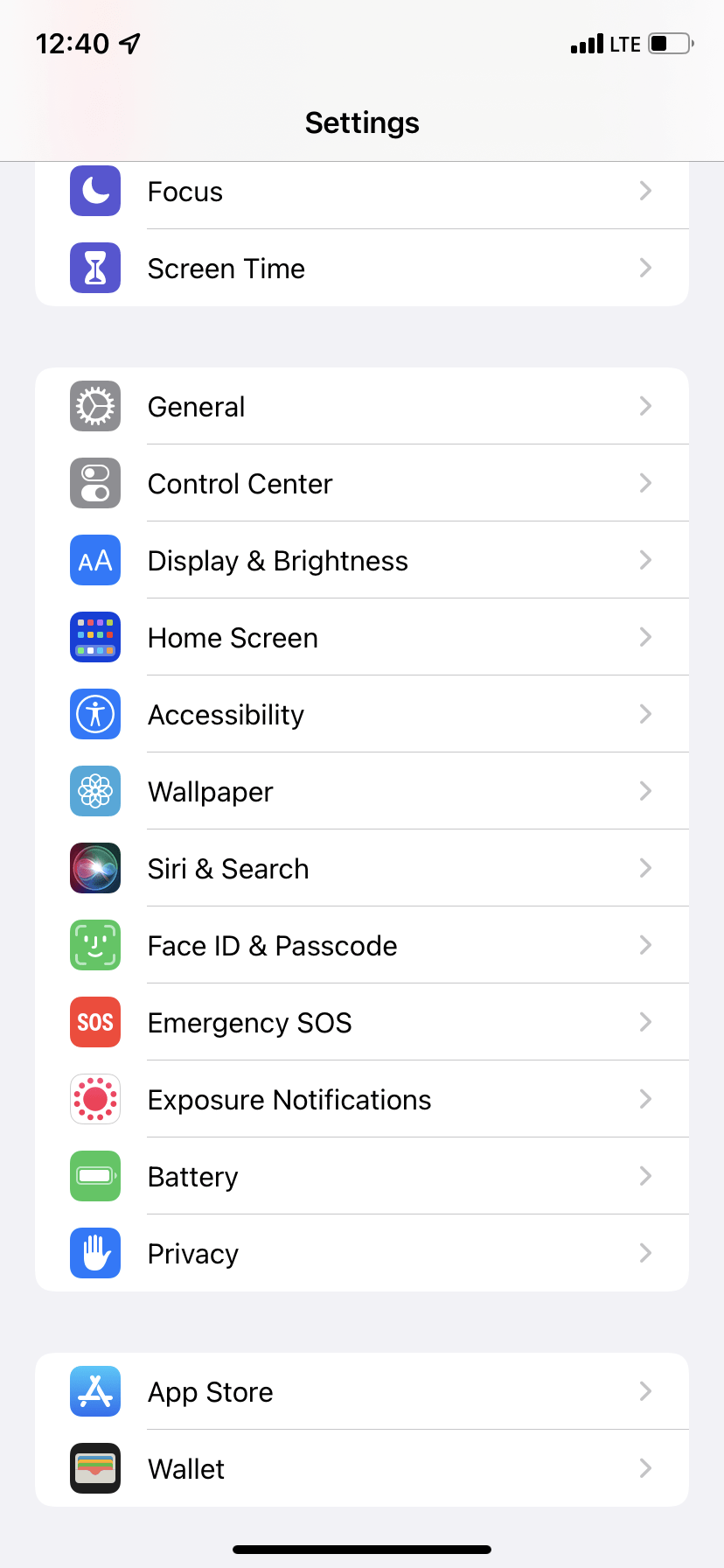The image displays an iPhone's Control Center interface, presenting a variety of settings and functionalities. The screen is not fully populated, indicating either customization or empty slots. Key features highlighted include the settings for Focus mode, screen time, and general controls. Prominently displayed are icons for Facebook, SOS emergency alerts, exposure notifications, battery status, and privacy settings. Additionally, the image shows multiple rows and icons, indicating a comprehensive range of options available. The App Store and Wallet apps are also visible. The search bar, tinted in gray, complements a distinct red square icon, adding a splash of color to the otherwise muted interface.